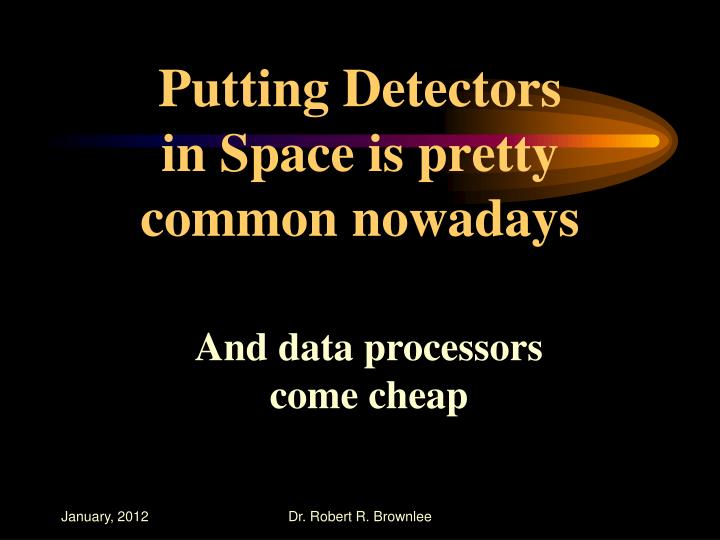The image features a black background, prominently displaying a comet or meteorite graphic extending from the left to the right. The comet transitions in color from deep blue through purple, ending in bright yellow-orange, with an impression of heat dispersion trailing behind it. Positioned at the top of the image, the text in vibrant yellow reads "Putting detectors in space is pretty common nowadays," while below, in smaller white font, it states "and data processors come cheap." At the bottom of the image, in small white text, it is dated "January 2012" on the left side, and centrally it reads "Dr. Robert R. Brownlee." This slide, resembling one used in a PowerPoint presentation, combines simple yet striking visual elements and essential information effectively.